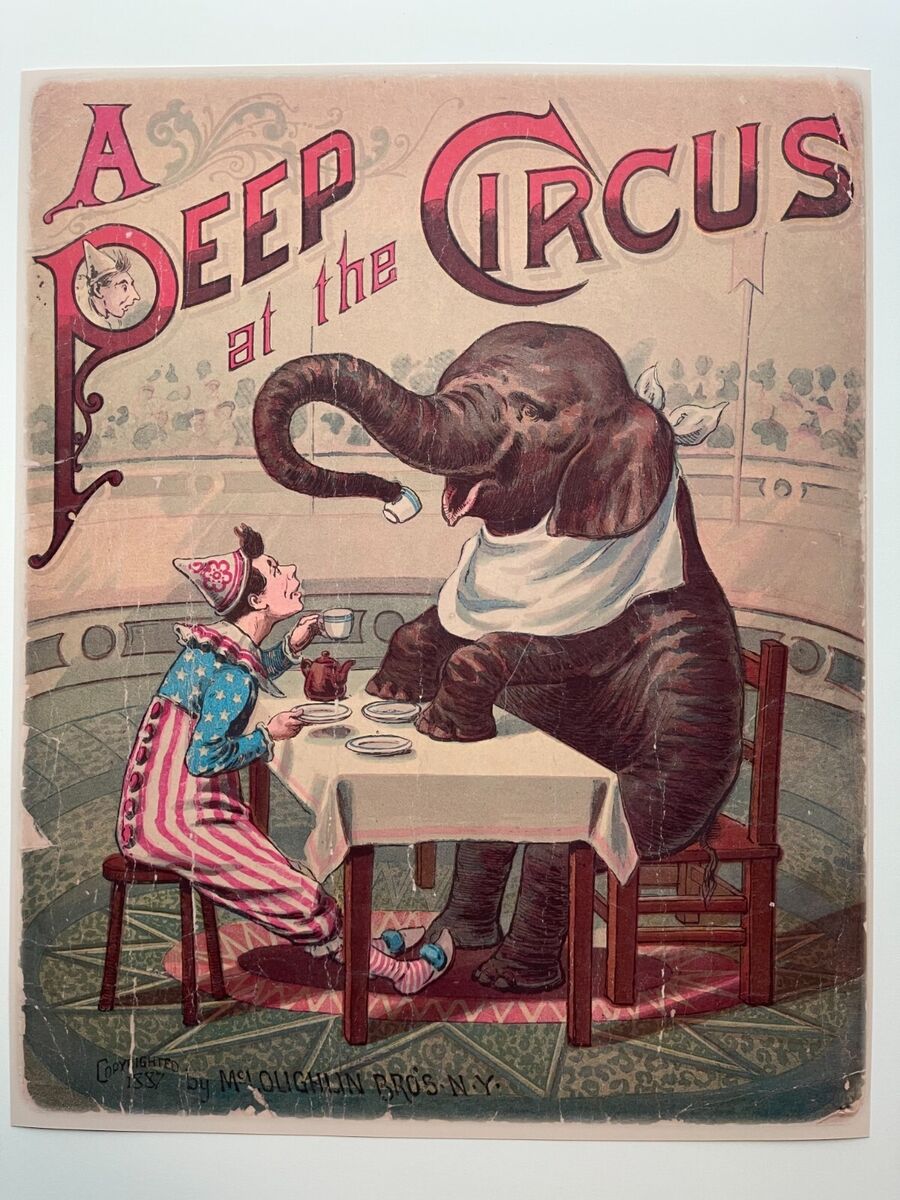This image portrays an old-fashioned poster advertisement titled "A Peep at the Circus" in bold red letters at the top. The scene illustrates a whimsical moment featuring a boy dressed in a clown suit, seated on a small wooden stool at a table, sharing tea with a smiling elephant. The wooden table, adorned with a white tablecloth, is set with a tea set, including cups resting on small dishes and a teapot. The boy holds a cup of coffee in his left hand while looking up, seemingly distracted by his unusual dining companion. On the other side of the table, the elephant, seated comfortably on a larger wooden chair, has a bib around its neck and is using its trunk to hold a teacup, ready to take a sip. The bottom of the poster credits its creation to McLaughlin Brothers, New York, and the entire image appears to be photographed against a light blue background.